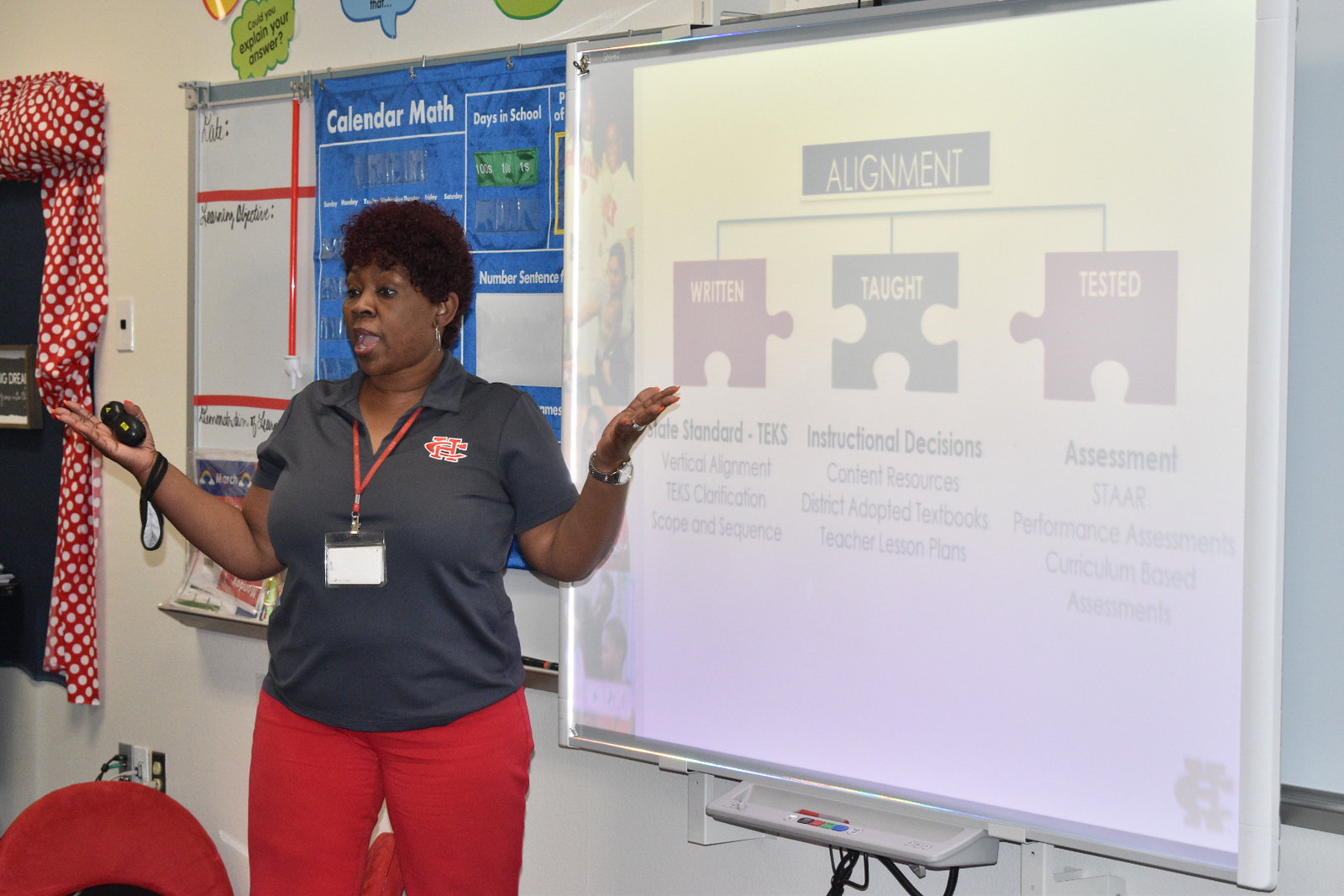In this horizontally oriented indoor photograph, a middle-aged African-American woman is presenting in a classroom setting. She has short dark hair with bangs and is speaking as she stands in front of a large white projection screen framed by a silver metal border. She is wearing a gray, short-sleeve, open-collar shirt, possibly a polo or knit shirt, with a logo resembling a "C" inside of an "H" on it, along with bright red pants. A red lanyard with a name tag hangs around her neck. Her arms are by her sides but bent at the elbows, with both forearms pointing upward as she gestures, and she holds a remote device in her right hand, likely to control the projector.

The screen behind her shows a faint image with a horizontal blue bar centered horizontally that reads "ALIGNMENT" in white capital letters. Below this bar, a diagram of three horizontal puzzle pieces can be seen, likely labeled "WRITTEN," "TAUGHT," and "TESTED." The leftmost piece appears red, the center blue, and the rightmost red. Each puzzle piece has faint white text, accompanied by bold lines of text and smaller paragraphs underneath, detailing components such as state standards, instructional decisions, and assessments.

To the left, a window is adorned with a red and white checkerboard curtain. Further along the white wall, a bulletin board displays indistinguishable items. Above the bulletin board, small, indistinct graphics in green and blue decorate the upper part of the wall near the ceiling. In the lower left corner of the photograph, a red, round object, potentially the back of a chair, is partially visible.